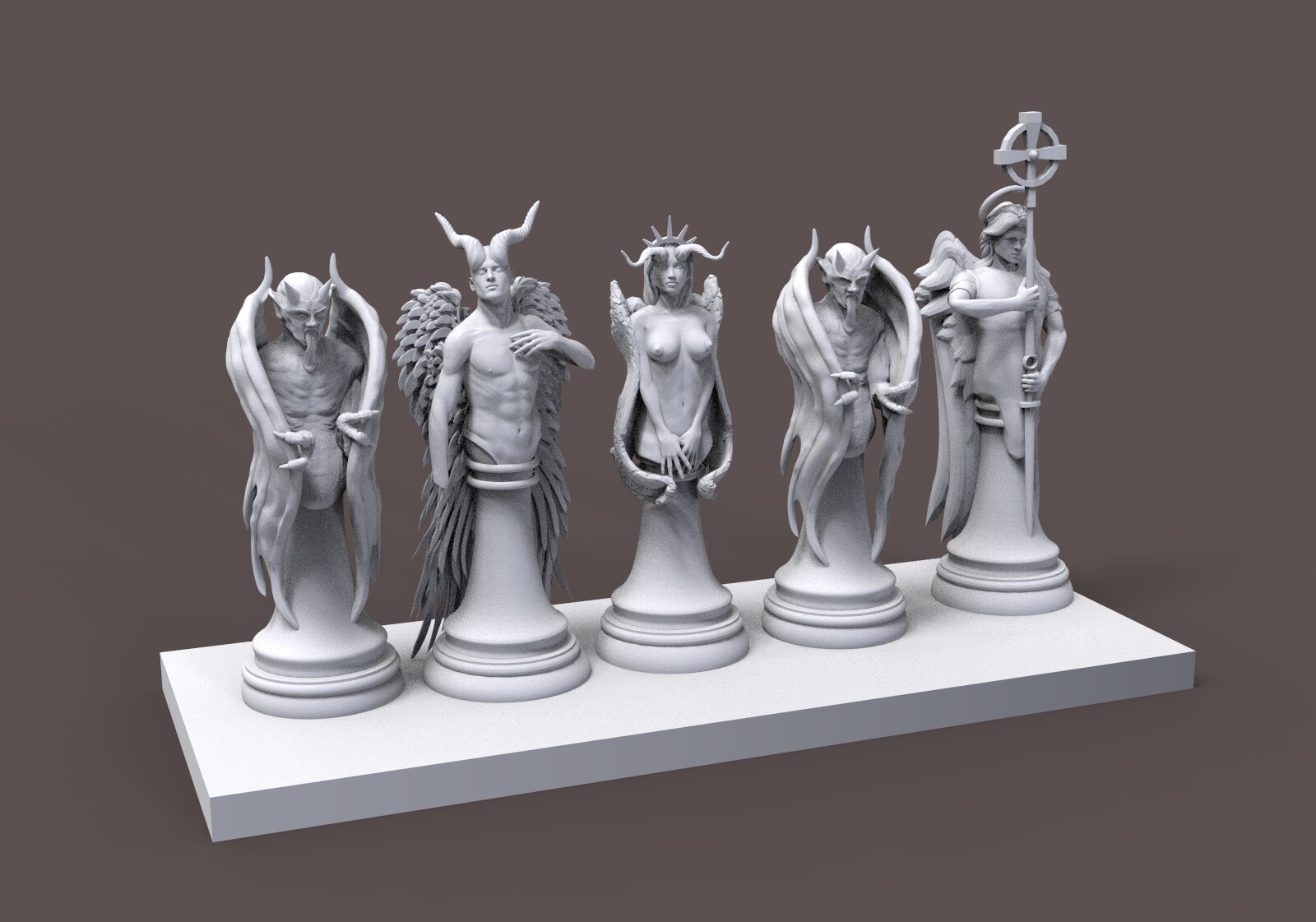The image features five intricately detailed figurines, lined up on what appears to be a digital floating shelf with a plain brown background. Each figure stands on a chess piece-like base and exudes an ominous, demonic presence. Starting from the left, the first figure resembles a devil, complete with horns, a small beard, wings, and talon-like fingers. The second figure has angelic, fluffy wings and sports long, curved horns. He holds his right hand near his heart, accentuating his muscular build. The third figure is a female with forward-pointing horns that tip upwards at the ends, a five-pointed crown reminiscent of the Statue of Liberty, and wings that wrap around her sides. The fourth figure is another devil-like entity, similar in appearance to the first figure. The final figure on the right holds a staff topped with a circle and cross and wears a halo. This figure also has wings extending behind them. The scene is hauntingly detailed, with each figure distinctly representing elements of angels, nudes, and devils, all set against a muted gray background.